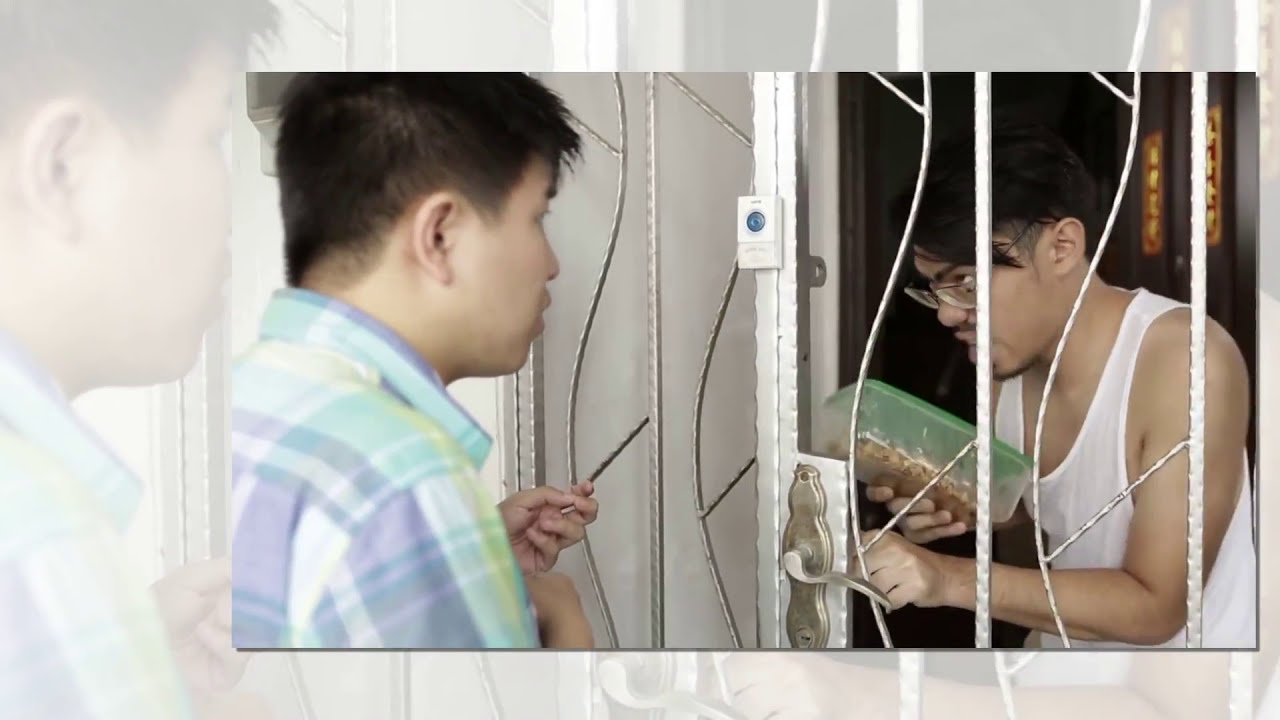This image captures a tense interaction between two Asian men at a front door. The man on the outside, positioned on the left, has short black hair and is wearing a pastel plaid button-down shirt. He appears to be gesturing animatedly, possibly in conversation or argument. On the right, separated by a silver wire metal door, the man inside the house wears glasses that sit low on his nose, a white tank top, and holds a green-lidded plastic container with an unknown contents. The man inside looks through the door with a stern, possibly angry expression, holding the door handle while engaging with the other man. The background features a mostly white wall accented with silver metal lines. The scene, marked by vibrant colors including blue, purple, yellow, green, black, tan, and gray, seems to unfold on a front porch, highlighting a vivid moment of human interaction.